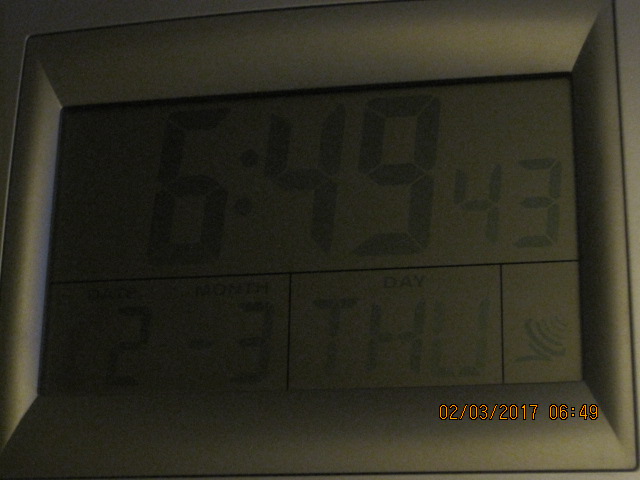This close-up image captures a square, metallic-gray digital clock in dark conditions, making the faint display somewhat difficult to see. The clock's display shows the time as 6:49 and 43 seconds, using a typical 7-segment digital readout. The date reads "Day 2, Month 3," confirming it's the 2nd of March, and the day is indicated as Thursday (THU). Additionally, there is a timestamp in the bottom right corner of the photo that reads 2-3-2017, 6:49. The clock display appears unlit, possibly due to low battery, and shows a symbol in the right corner, resembling slashes, which might indicate a wireless function. Overall, the photograph focuses mainly on the clock's display without revealing the entire device.